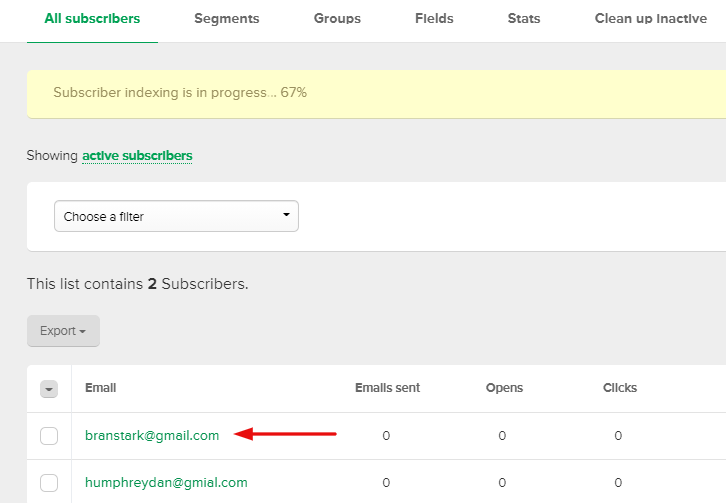In the top left corner of the image, the phrase "All Subscribers" is displayed in green and underlined in the same color. To the right, there are several options listed: Segments, Groups, Fields, Stats, and Clean Up Inactive. Below this array, a light yellow notification box states, "Subscriber indexing is in progress, 67%." 

Beneath this, the word "Showing" appears above "Active Subscribers," which is also in green and underlined. Below this header, a dropdown box labeled "Choose a filter" with a downward-pointing arrow is visible. 

The list reveals that there are two subscribers, with the number "2" highlighted in black. Below this count, an "Export" button is positioned inside a separate box.

Descending further, an email section appears. The heading "Email" is followed by the email "brenstark@gmail.com" in green, which is marked with a red arrow pointing towards it for emphasis. Below this email address, "humphreydan@gmail.com" is listed.

Next to the "Email" heading, three columns outline further subscriber details: "Emails Sent," "Opens," and "Clicks."